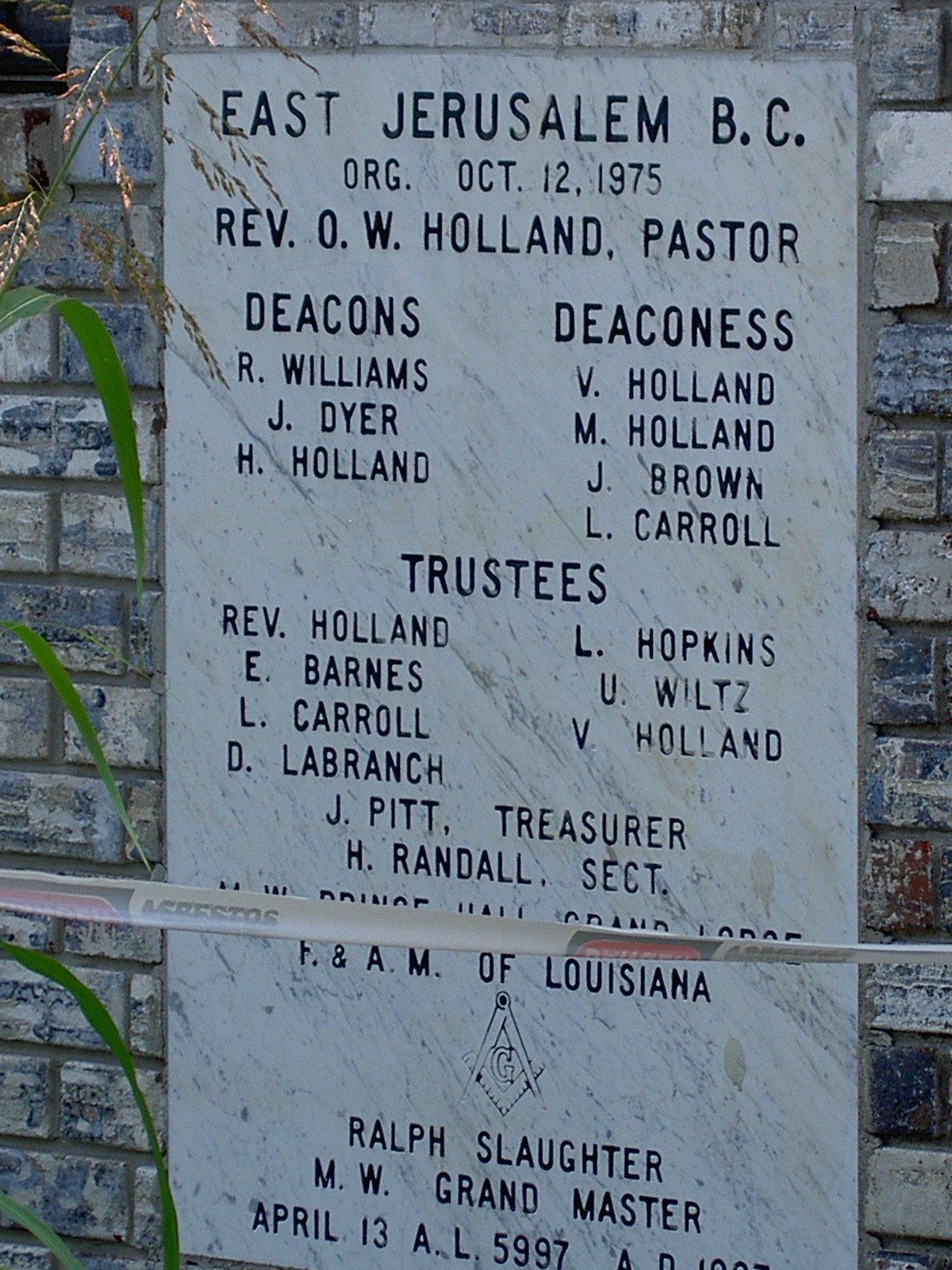The image depicts a white marble plaque, set into a red brick wall, with subtle discoloration in shades of gray and brown. The plaque is inscribed with several sections of text, arranged meticulously in columns. At the top, the plaque reads "East Jerusalem BC," followed by the date "October 12, 1975." Below that, it lists "Rev. O. W. Holland, Pastor," and provides a detailed roster of deacons and deaconesses. Further down, there is a section dedicated to trustees, presenting a comprehensive list in two columns. At the bottom of the plaque, it reads "Ralph Slaughter M.W. Grandmaster," noting an additional date, April 13th, Al-5997. The scene also includes some foliage, with bushes visible on the left side of the photograph, adding a touch of greenery to the setting.